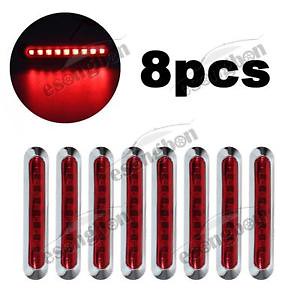This advertisement image showcases a set of red LED lights, specifically 8 pieces neatly aligned from north to south at the bottom of the image. Each light has a shiny silver exterior with a red-tinted lens and approximately ten LEDs inside. The image illustrates the lights standing upright, resembling thermometers with their oblong shape, red middle, and chrome-like appearance. At the top left corner of the image, a black circle depicts one of these lights turned on, emitting a red glow that reflects off the surface, illustrating its illumination in the darkness. Bold black text to the right of this circle prominently indicates "8 PCS." Additionally, there's a faint, difficult-to-read watermark, possibly spelling out "E-S-O-N-G-B-O-N-S" or another brand name.